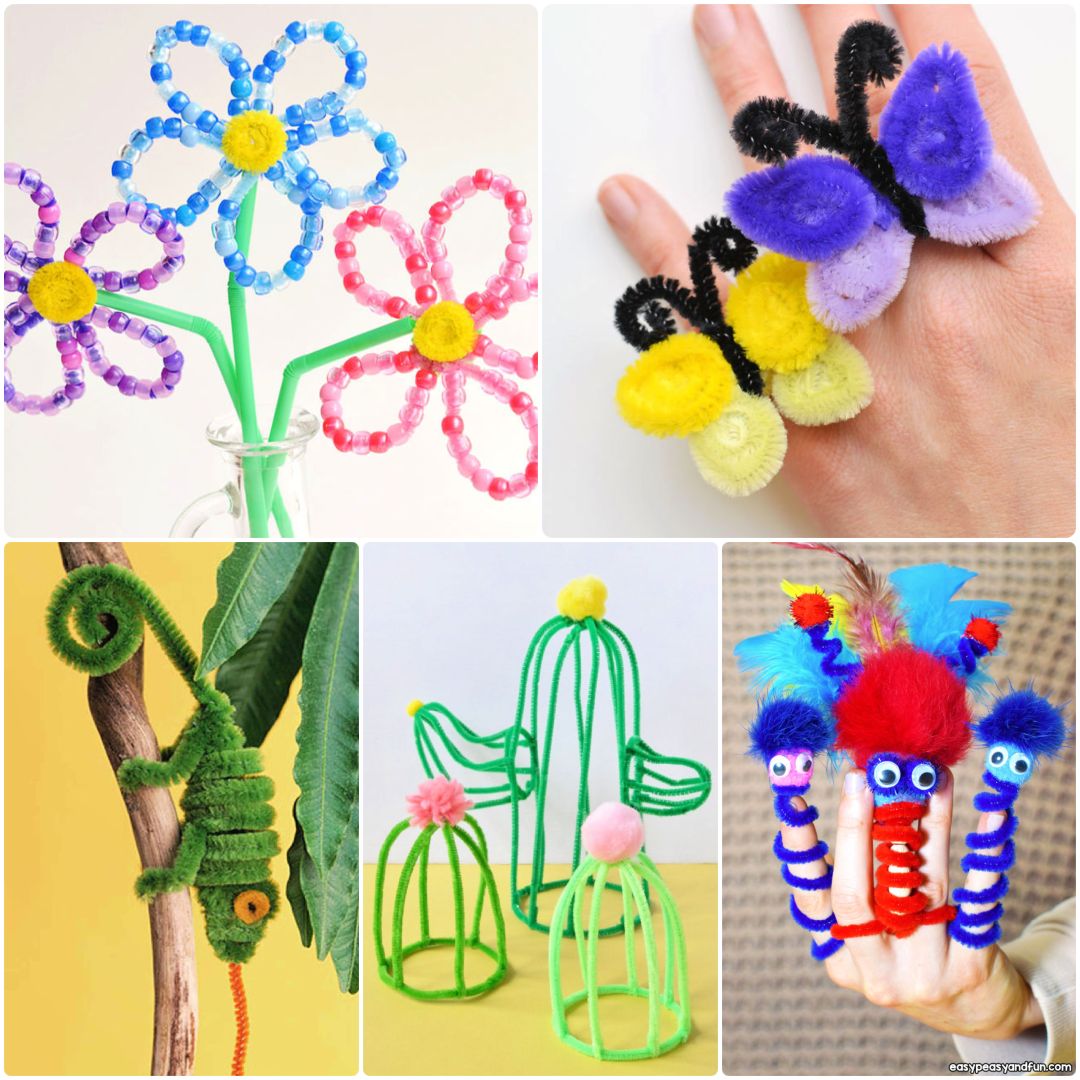The image is a collage showcasing five hand-made crafts. In the top left corner, three colorful straw flowers with green stems are arranged in a clear glass jar; the flowers' blooms are blue, purple, and pink with yellow centers. Directly to the right, two fuzzy butterfly rings crafted from pipe cleaners are displayed against a backdrop; the butterfly on the left is yellow with a black center, while the one on the right is blue and purple with a black center and antennae. The bottom left corner features a vibrant green gecko made of pipe cleaners, with yellow eyes and a red tongue, clinging to a brown wooden branch with green leaves beside it, all set against a yellow background. The bottom center image showcases intricate straw bird cages, with three cages on display. Finally, the bottom right image presents a woman's hand wearing several finger puppets, predominantly blue and red, with strings wound around her fingers. The overarching theme of this collage is creative, home-made crafts, each piece showcasing unique materials and imaginative designs.